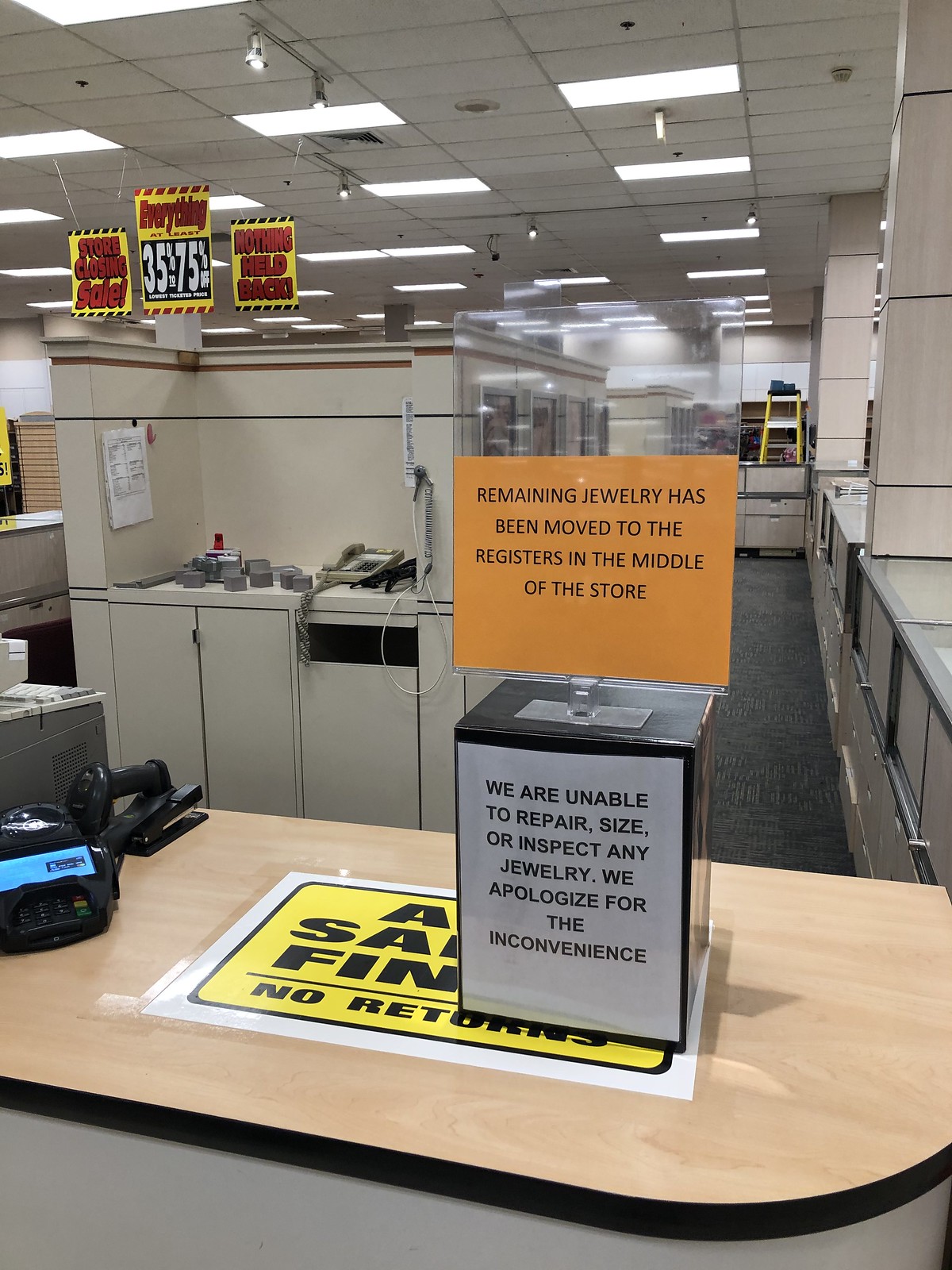This photograph depicts the interior of a retail store, potentially a former Kinko's, office furniture sale outlet, or a bedroom furniture sale store. Prominently displayed at the forefront is a sign informing customers that all remaining jewelry has been relocated to the register area in the middle of the store. The notice also states that the store is unable to repair, size, or inspect any jewelry and apologizes for the inconvenience. This policy may have been implemented due to previous issues, possibly involving theft or disputes over jewelry repairs. 

In the same vicinity, another sign on a desk clearly states, "All Sales Are Final, No Returns." Resting on that desk is a black phone, a black scanner, and a cash register. Nearby, additional signs announce significant discounts of 35% to 75% off on various items, with a note declaring "Nothing Held Back." The overall atmosphere suggests a clearance sale or liquidation event, marked by persistent reminders of final sales and substantial price reductions.